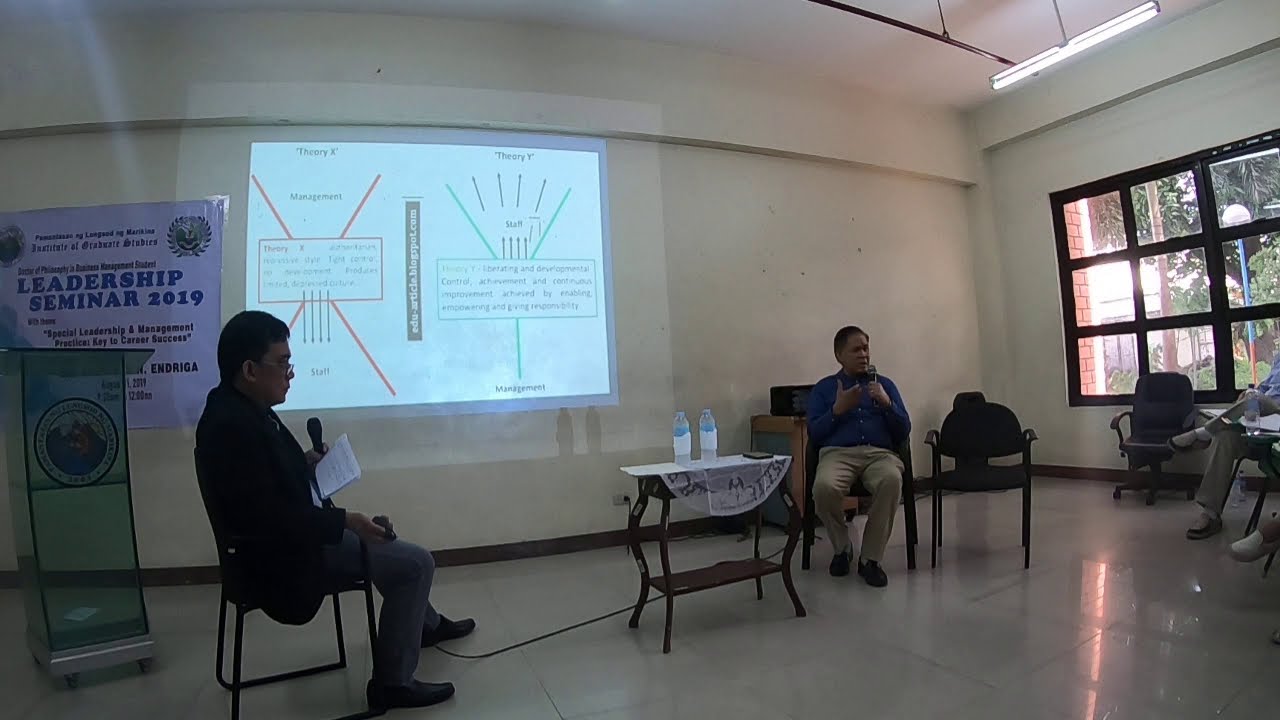The photo captures an indoor seminar setting, identified as the "Leadership Seminar 2019" by a prominent banner at the back. The room is dimly lit, suggesting a focus on the presentation. Central to the image are two speakers situated at a table that has water bottles on it. Both speakers appear to be presenting, using microphones, with one person positioned slightly to the left and closer to the viewer, likely the host, while the other speaker, perhaps the main guest, is to the right. Behind them, a projector displays content on two different theories. The setting resembles an educational environment, possibly a classroom, with a tile floor visible at the bottom of the image. Additional details include a window on the right side of the room, a few visible attendees seated and listening attentively, and varied colors present throughout the scene, including white, green, black, red, blue, orange, gray, and light blue. The image captures a professional atmosphere in the middle of the day, with focused interaction between the presenters and the audience.